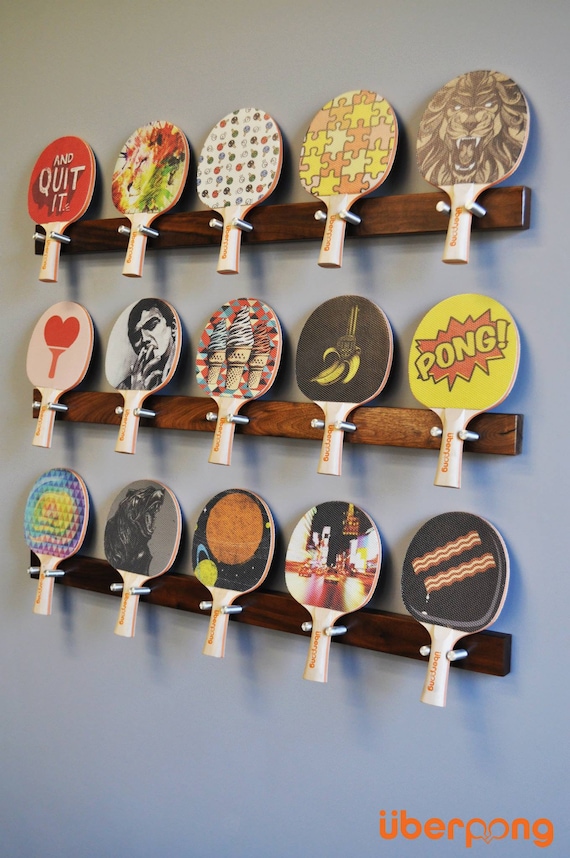This photograph captures an artistic wall display of fifteen uniquely designed table tennis paddles organized in three rows of five, each row mounted on a brown wooden bar supported by silver metal pegs. The paddles, all from the same brand, feature a variety of vibrant and diverse designs against the backdrop of a gray-blue wall. Among the standout designs, there is a paddle with the text "QUIT IT" in the top left, a striking image of a roaring lion, a jigsaw puzzle pattern, and a whimsical illustration of a banana revealing a gun. Additionally, there are paddles adorned with paint splatters, ice cream cones, a heart-shaped paddle, slices of bacon, and a black-and-white depiction of a man's face, possibly Johnny Cash. The bottom right of the display prominently features an orange logo reading "Uber Pong." The illumination from the left casts distinct shadows to the right, enhancing the visual depth of the display. The paddles appear to be machine-printed, contributing to their uniformity in craftsmanship while showcasing their unique decor.